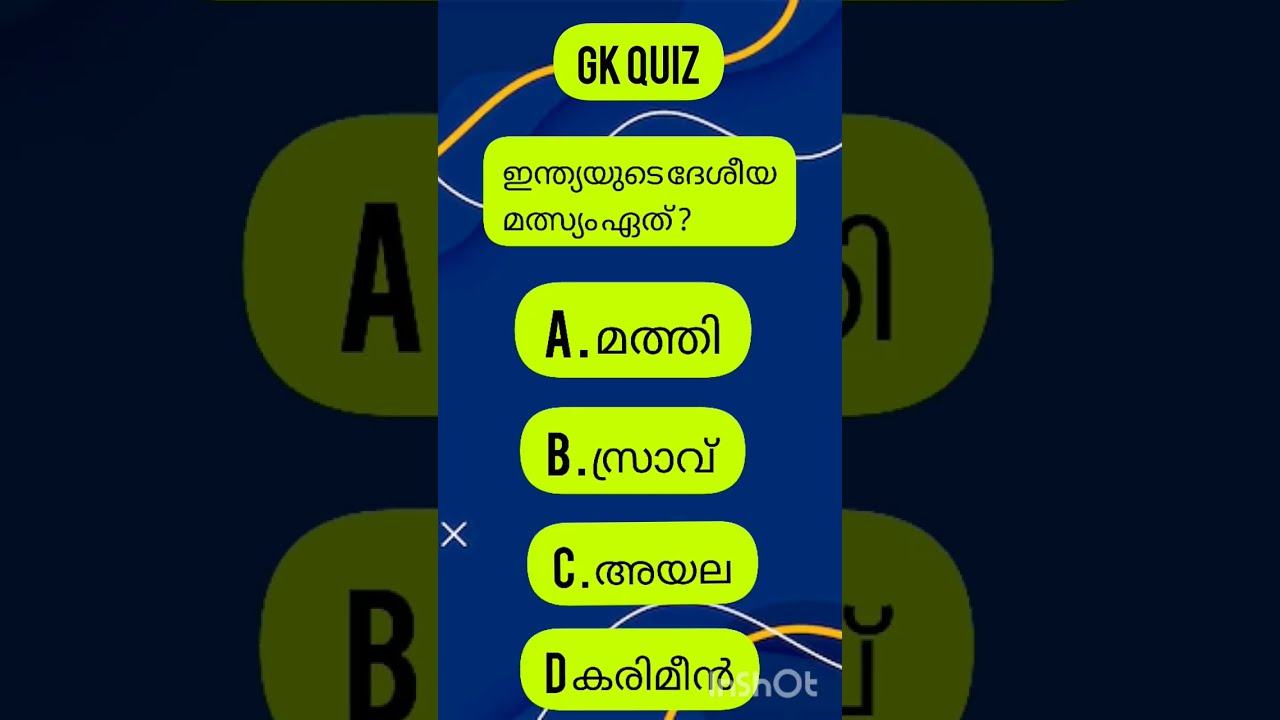The image features a detailed, multi-layered design that consists of a central, vertically-aligned picture with a faded, zoomed-in version of the same image in the background, filtered darkly on its sides. At the core is what seems to be a cell phone app interface, showcasing a "GK quiz" title in bold, black text on a lime green, oval-shaped rectangular background. Below the title, there is a quiz question written in a foreign language characterized by curvy lines, also laid out on a matching lime green background with rounded corners. The question is followed by four answer choices labeled A, B, C, and D, with each option's text differing slightly in length, particularly the choice labeled 'D,' which is longer. The entire arrangement is set against a striking blue background adorned with abstract yellow patterns, vibrant orange and white wavy lines, which add an additional layer of visual intrigue. The central image spans approximately 7 to 8 inches in width and 5 inches in height, and the overall quality of the image is decent, making the text and patterns clearly visible.